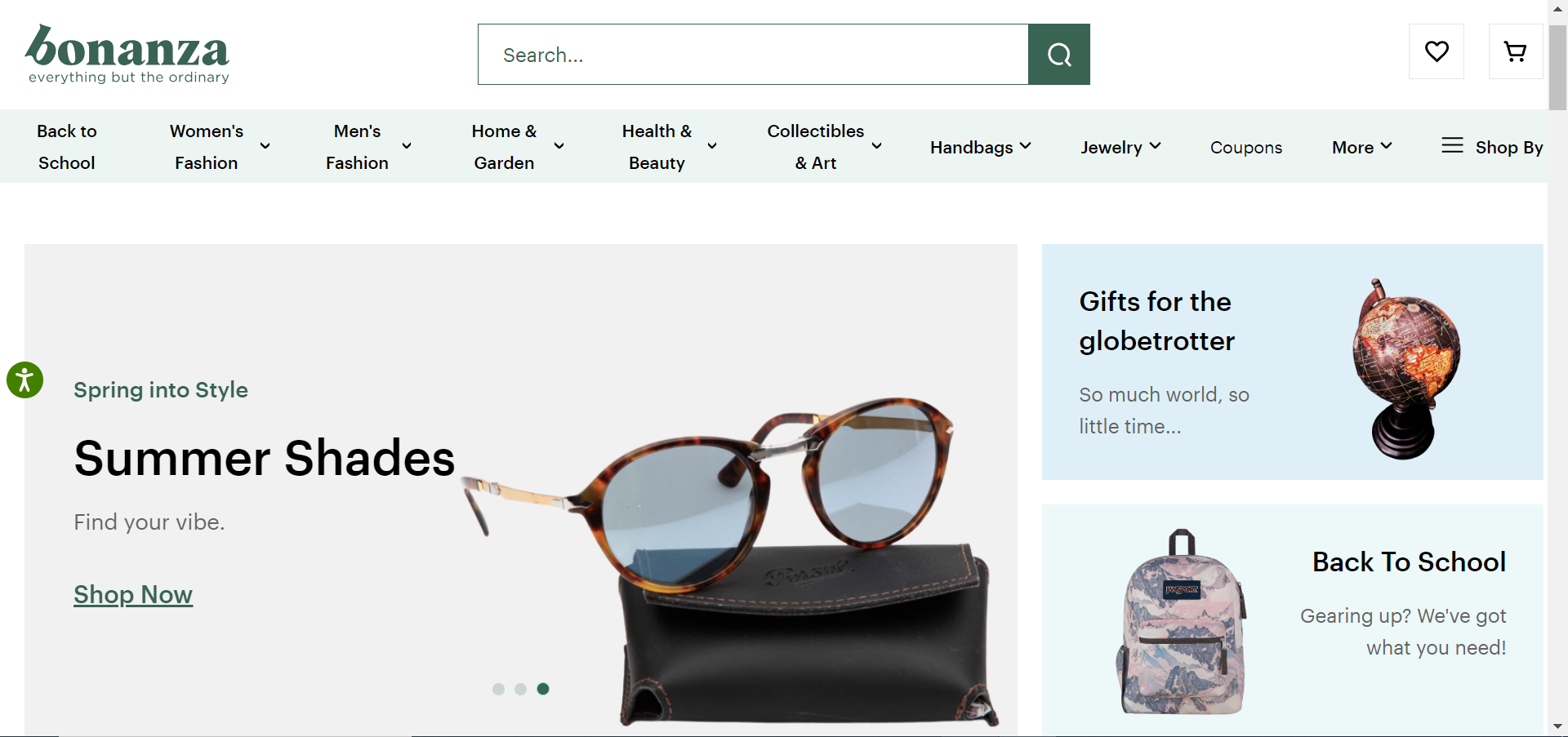This image showcases the Bonanza web page, a platform characterized by its tagline, "Everything but the ordinary." The Bonanza logo, prominently placed on the left side of the page, is rendered in green. Immediately below the logo, the tagline is displayed.

At the center top of the web page is a search box, with the prompt "Search" visible within it. To the top right, there are two clickable options: a 'Favorites' icon represented by a heart, and a 'Cart' icon. Both icons are enclosed within squares for easy accessibility.

Beneath these options is a navigation bar featuring various clickable links. From left to right, the links are: "Back to School," "Women's Fashion," "Men's Fashion," "Home and Garden," "Health and Beauty," "Collectibles and Art," "Handbags," "Jewelry," "Coupons," and "More." Following this list is a "Shop By" button.

The section below this navigation bar features promotional content. The first promotional image is titled "Spring into Style," "Summer Shades," and "Find Your Vibe, Shop Now," and showcases a picture of summer shades. Adjacent to this, on the right, is an advertisement labeled "Gifts for the Globetrotting," accompanied by an image of a globe and the caption, "So much world, so little time."

Finally, below these advertisements is another promotional section titled "Back to School," with the sub-heading "Gearing up, We've got what you need." This section includes an image of a Jamesport book set.